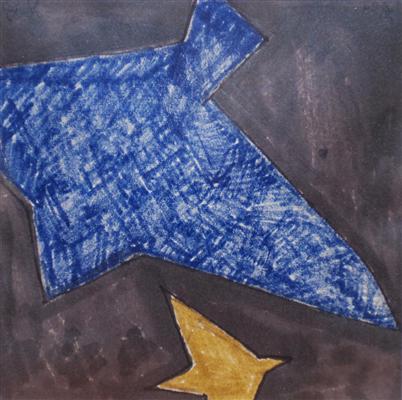The image is a child's painting with a dark, muddy purple or black watercolor background. Prominently featured is an irregular, solid blue shape with angular, sharp edges that resembles a fish with fins but could also be interpreted as a bird. This blue shape appears to be filled in with marker, showing some faded criss-crosses and white patches where the color is incomplete. Below it is a smaller, irregular yellow-orange shape, which also resembles a bird in flight. The blue shape is large and central while the yellow-orange shape is small and positioned towards the bottom of the painting. The overall artwork has a rudimentary, childlike quality with basic coloring techniques and simple shapes.